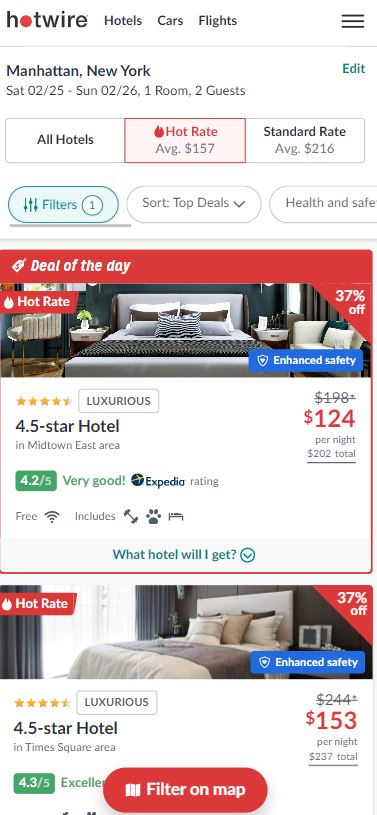The website interface for Hotwire is displayed prominently, with the brand name "Hotwire" in black text, except for the 'O' in "Hot," which is stylized as a red circle. Directly below, black text indicates available services: "Hotels," "Cars," "Flights," accompanied by a three-bar menu icon on the right.

A thin gray line spans the width of the page, beneath which date and location details are provided: "Manhattan, New York, Saturday 02/25 to Sunday 02/26, One Room, Two Guests." To the right of this information are "Edit" and "Change" options.

Three category banners are listed:
1. "All Hotels" in black.
2. "Hot Rate" styled with a light red background, red text, and small red flames, noting an average price of $157.
3. "Standard Rate," marked with an average price of $216, formatted in classic text.

Below these, several filter options appear as oval buttons:
1. "Filters" with a green background and text, containing a white circle outlined in green with the number 1 inside.
2. "Sort" next to "Top Deals," indicating filters or arrangements.
3. "Health and Safe."

A "Deal of the Day" section appears on a red banner declaring "37% off." An image of a hotel bedroom is provided, displaying the text "Hot Rate" on a red banner, alongside a blue banner stating "Enhanced Safety," and a description as a "Luxurious 4.5-star hotel" with gold stars visible. Location details include "Midtown East Area," with the original price of $198 crossed out and a new price of $124 in red. Additional information includes a description "Per Night, $202 Total," a green banner rating the hotel at "4.2 out of 5, Very Good" in green text, and a blue "Expedia" logo. Icons for free Wi-Fi, a pet paw, and a bed are shown, followed by a green inquiry, "What hotel will I get?" with a downward-pointing arrow.

The next listing mirrors the format:
- "Hot Rate" on a red banner.
- "37% off" in white text against red.
- "Enhanced Safety" on a blue banner.
- Gold stars indicating a "4.5-star hotel in Times Square."
- Price details with an original rate of $244 crossed out and a new rate of $153 in red.
- Information on total cost: "Per Night, $237 Total."
- A green banner stating, "4.3 out of 5, Excellence."

At the bottom, a red banner with "Filter on Map" in white text completes the page.